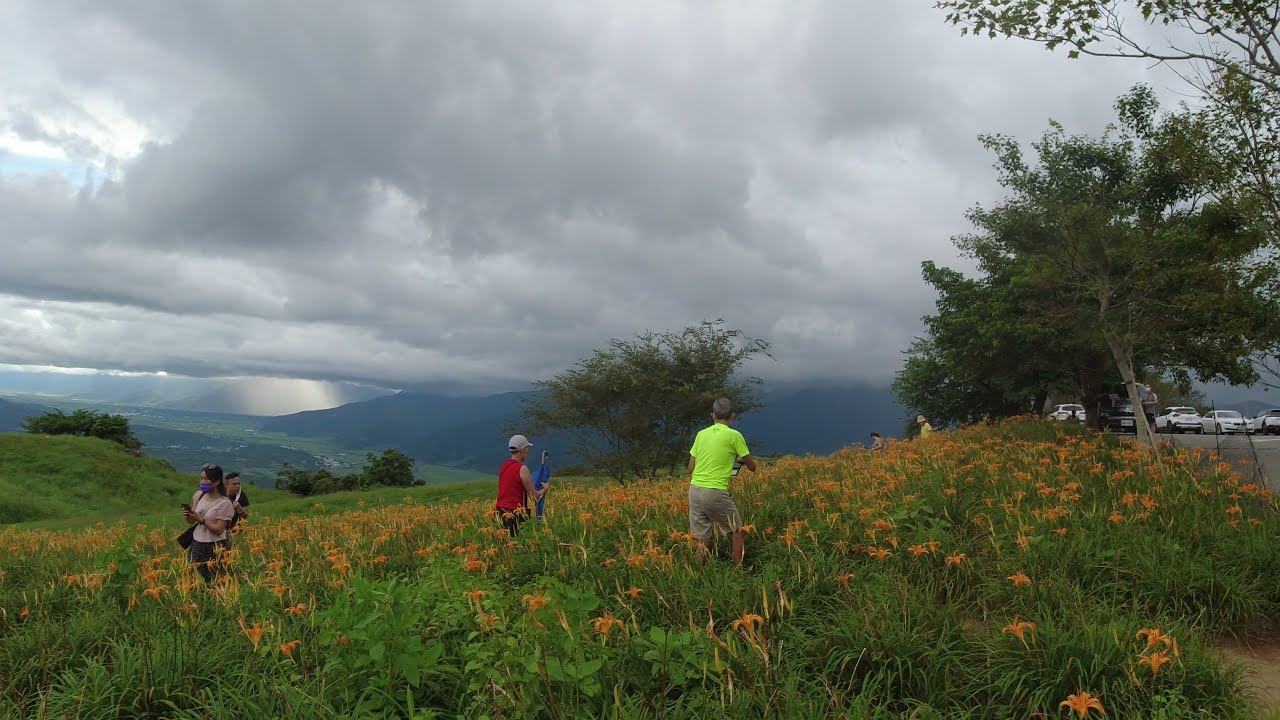The image captures a group of four people standing in a lush, green field filled with vibrant orange daylilies, set against the backdrop of towering mountains. The field appears to be knee-high with a mix of grasses and flowers. The sky is dominated by dark, foreboding clouds with patches of blue, suggesting either an impending storm or the aftermath of rain, as distant rainfall can be seen. 

The group of four is prominently in the foreground. The person in front, with their back to the camera, is a man wearing a neon yellow shirt and khaki shorts. Next to him is someone in a red sleeveless shirt, a ball cap, and carrying a blue umbrella. Facing the camera, somewhat indistinct, is a couple—a man and a woman. Off to the far left, partially visible, is a person in a white shirt with dark pants, possibly wearing a blue COVID mask. A black-shirted individual stands behind them, and another person in a red shirt, black pants, and a white hat is close by.

In the background, on the right edge of the image, a parking lot with mostly white cars and one black car—or possibly a dumpster—can be seen. This lot is separated from the field by a line of green trees. Beyond the lot, a body of water gleams faintly in the distance. The hills transition smoothly into the dense green of the mountainous terrain, adding to the scenic beauty of this outdoor landscape.